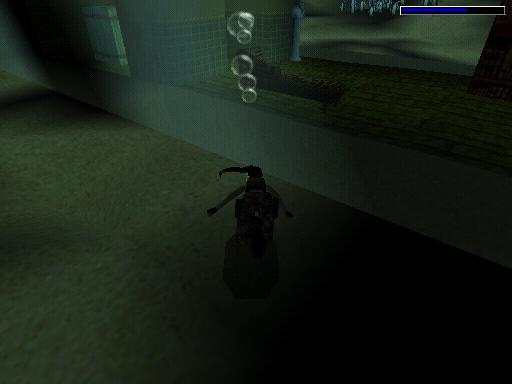In this still frame from a dark, older video game, a central character is depicted running on what appears to be dark green or concrete ground. The scene is predominantly dark gray and black, emphasizing a mysterious ambiance. The character, seen from behind, seems to be wearing a dress with a backpack and has a ponytail braid extending to the left. Both of their arms are outstretched. Shadows obscure much of the detail, but faint, glowing eyes can be discerned on the character. Three white bubbles float upward from the character, further adding to the eerie atmosphere. To the right, a gray section features more bubbles rising from it. There is a grassy or ledged ramp descending and ascending nearby, hinting at navigable terrain. In the top right corner, a thin rectangular bar with a blue section, approximately two-thirds full, might be indicating the character's health or stamina. Beyond the ledge, there appears to be a darker area, possibly a room or another part of the building, with indistinct shapes suggesting furniture or creatures. The background gradients from blue to gray, creating a surreal and shadowy environment.